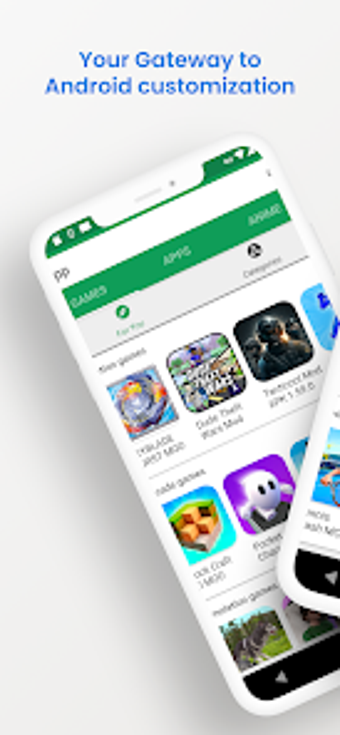The top section of the image features a blue, two-line text over an off-white background. The first line reads "Your Gateway" with capitalized 'Y' and 'G', and the second line reads "TO Android" with 'TO' capitalized and 'Android' in capital letters. Below this blue text, the word "Customization" is displayed, spelled out as "C-U-S-T-O-M-I-Z-A-T-I-O-N".

The main element in the image is a smartphone positioned diagonally, its bottom edge cut off, revealing a white search box at the top with the text "Black PP". Below the search box, there are tabs with green backgrounds labeled "Games" and "Apps". The text in the third tab is blurry and unrecognizable. Beneath these tabs are various icons and categories depicted in a mixture of colors, such as red, blue, black, white, purple, orange, and green. Some recognizable elements include a white ghost on a purple background and a section labeled "Ad Games", though much of the text remains unreadable due to the blur.

Adjacent to the main phone is the bottom left corner of another phone, barely visible, showing only its black base and white outline. The screen of this secondary phone displays a white triangle pointing downward, set against a black background with illegible text. The partially visible image on this phone depicts a white hand gripping a silver bicycle handle, surrounded by what appears to be white water, rocks, and green plants, giving an animated appearance.

This image captures the vibrant interface of an Android device, emphasizing customization options and various app categories, while partially displaying an animated scene on a secondary device.